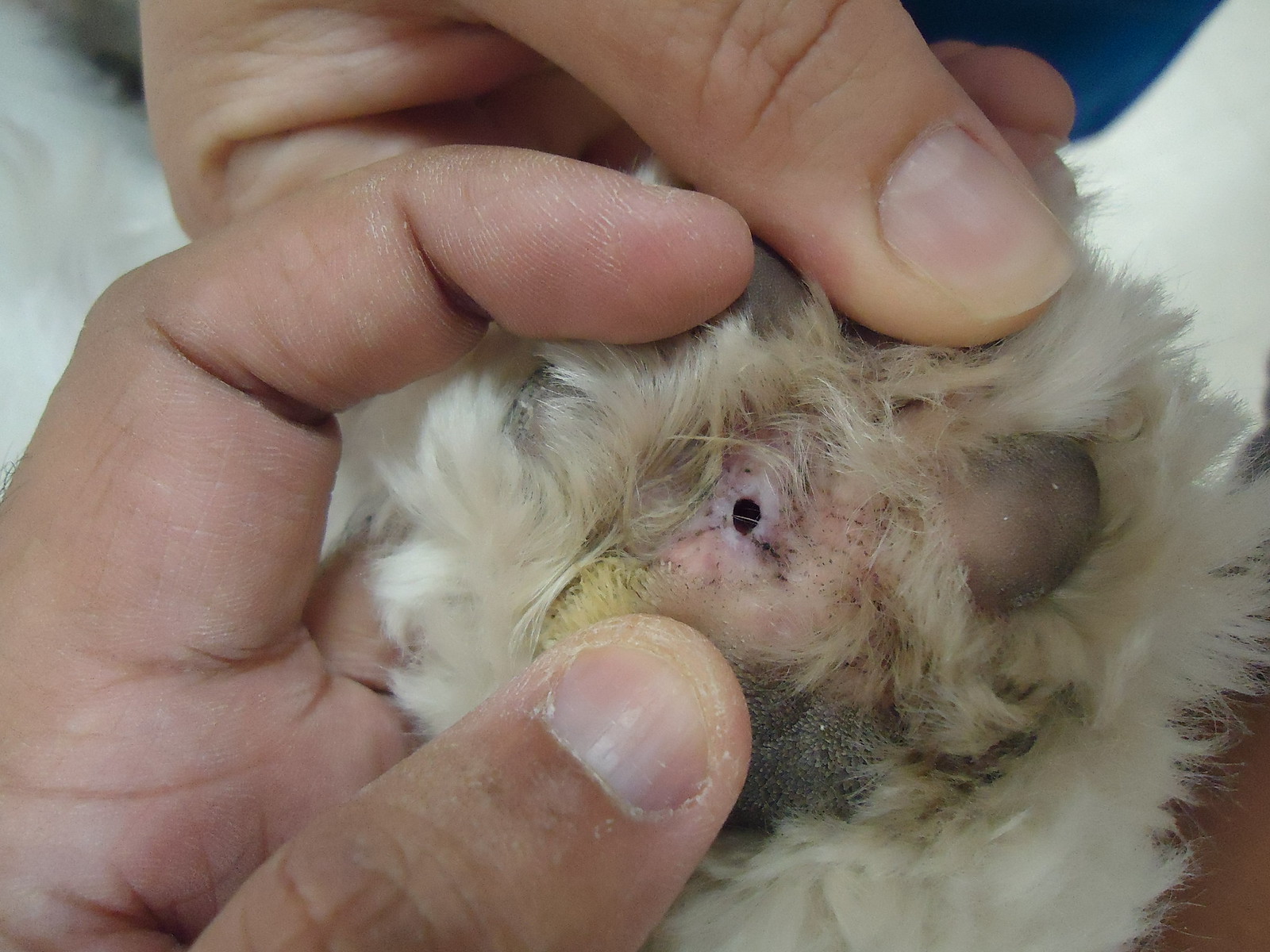In the image centered on a white countertop adorned with a blue mat, two human hands meticulously part the fur on a creature's paw, revealing the delicate anatomy. The fur, primarily white with hints of blonde, frames a paw that is predominantly pink and edged in black. One side of the paw exhibits a troubling yellow discoloration, and the flesh displays a conspicuous injury: a black hole encircled by stark white skin, indicative of significant trauma. The surrounding area is peppered with black specks. The hands, captured in fine detail, show dry fingertips and nails trimmed back to the quick. Despite the angle obscuring a clear view of the creature, the photograph conveys a sense of urgency and care in addressing the injury.